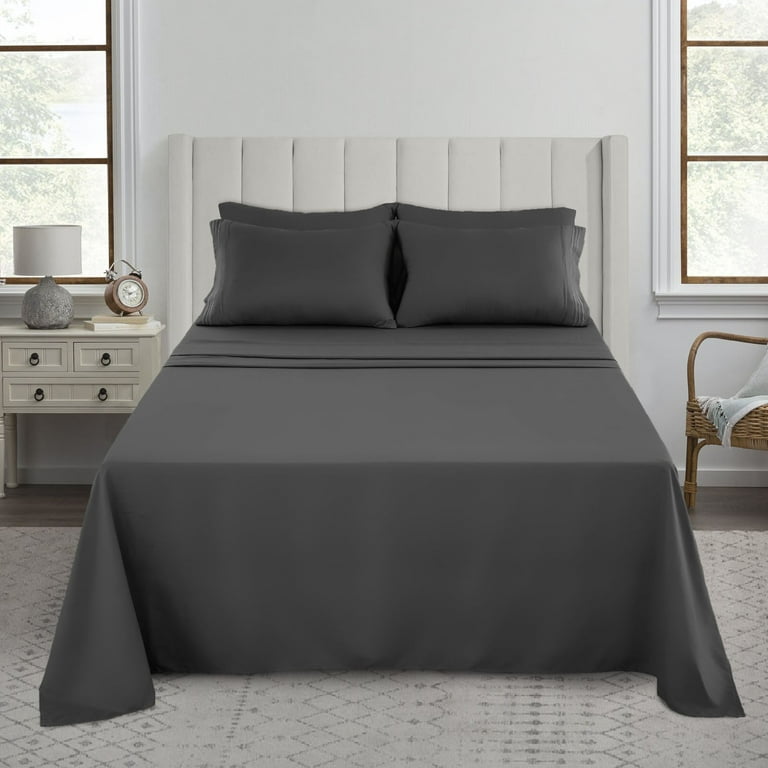This photo depicts a meticulously arranged bedroom with a formal aesthetic. The bed, adorned with four neatly placed gray pillows against a large, cushioned white headboard, features a perfectly folded gray sheet. On the floor lies a light gray, predominantly white carpet patterned with a diamond design. To the left of the bed stands a small white nightstand with multiple drawers, topped with an old-fashioned circular alarm clock and a lamp. The right side of the bed features a wicker chair draped with a blanket. The room has partial views of two windows, one to the left and another to the right, both providing a glimpse of outdoor trees through brown window sills. The overall atmosphere is neat and serene, amplified by the clean lines and orderly arrangement.